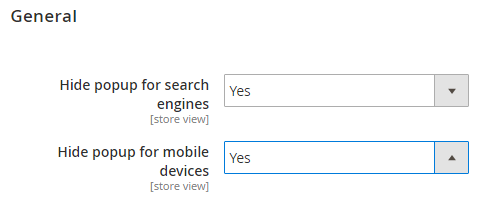This image is a screenshot from the settings page of a web application or content management system, under a section titled "General." The page features two specific settings, each accompanied by a drop-down menu for selecting options. The first setting is labeled "Hide Pop-up for Search Engines," and the selected option for this setting is "Yes." This implies that any pop-up elements such as notifications, advertisements, or messages will be hidden from search engine crawlers. By enabling this setting, the website aims to enhance its SEO performance by preventing these potentially intrusive elements from affecting its search engine rankings. Pop-ups are often viewed negatively by both users and search engines, as they can interfere with the user experience and diminish the site's attractiveness. By choosing to hide these pop-ups, the website is likely striving to present a cleaner, more user-friendly interface that avoids the pitfalls of intrusive pop-ups.